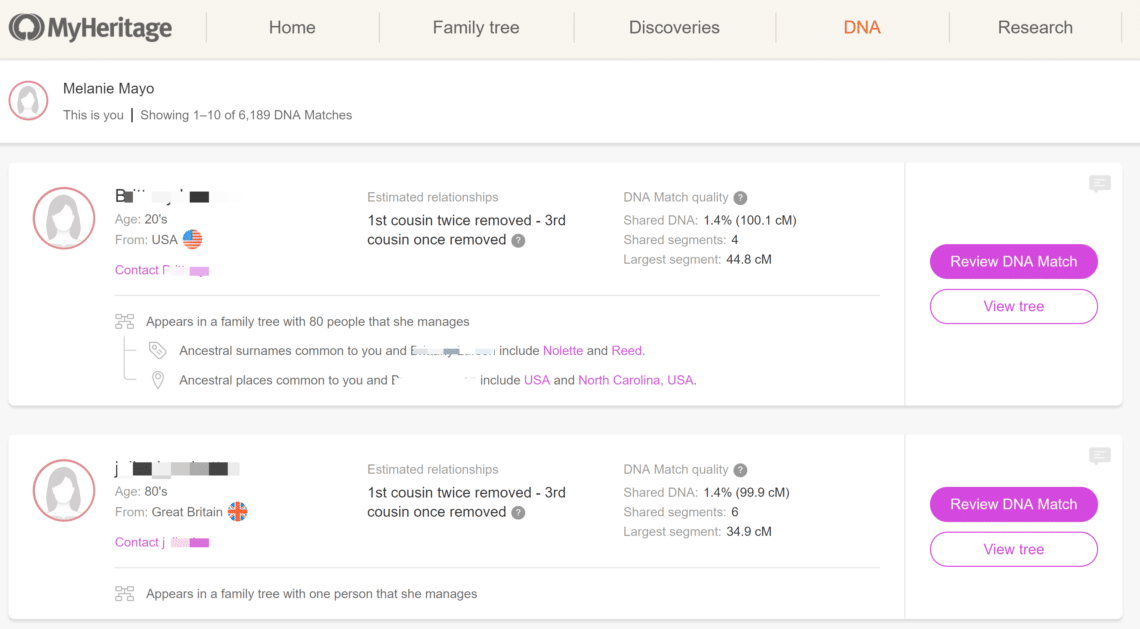This screenshot captures the MyHeritage website interface, specifically highlighting the DNA matches section. At the top of the website, there is a navigation bar featuring options such as "Home," "Family Tree," "Discoveries," "DNA" (selected), and "Research." The user's name displayed is Melanie Mayo, indicated as "This is you."

The screenshot presents DNA matches, displaying records 1 through 10 out of 6,189 total matches. For the first DNA match, details provided include:
- Estimated relationship: First cousin twice removed or third cousin once removed.
- DNA match quality: Shared DNA at 1.4%, with four shared segments and the largest segment measuring 44.8 centimorgans (cm).
- Options: "Review DNA match" and "View the tree."
- Additional info: The person is estimated to be in their 20s and located in the USA. They appear in family trees managed by Melanie Mayo, with ancestral connections to the USA and North Carolina, and surnames Nullet and Reed.

The second DNA match shows:
- Estimated relationship: First cousin twice removed or third cousin once removed.
- DNA match quality: Shared DNA at 99.9%, with six shared segments.
- Options: "Review DNA match" and "View the tree."
- Additional info: The person is estimated to be in their 80s and is located in Great Britain.

Overall, this detailed view highlights the familial connections, DNA match quality, shared segments, and options for further investigation into the family tree, underscoring the engaging exploration of ancestral ties.